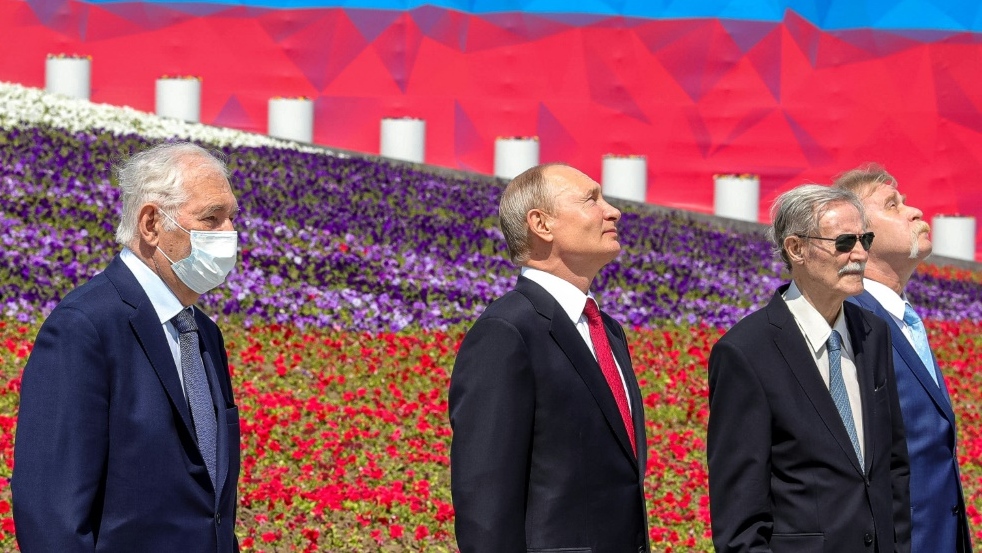In this image, four well-dressed politicians, all in suits and ties, stand together. The oldest among them, positioned at the far end, is notably wearing a mask covering his mouth and nose. The second man from the left closely resembles Vladimir Putin, the President of Russia, and could likely be him. The man beside Putin, on his right, is wearing glasses. Each man appears to be of an advanced age, with Putin seemingly the youngest among them. They are all gazing upwards, particularly Putin and the man with glasses. 

Behind them is a visually striking array of flowers: a first row of vibrant red flowers, followed by fields of purple and white blooms. The background, however, features an enigmatic red and blue backdrop that suggests an indoor setting despite the lifelike appearance of the flowers, which could be part of a painted scene or a mural. This adds an element of uncertainty about whether the picture has been digitally altered or if it was taken in an unusually picturesque venue. Despite these ambiguities, the four men maintain a poised and formal demeanor, contributing to the overall impression of a highly orchestrated event.